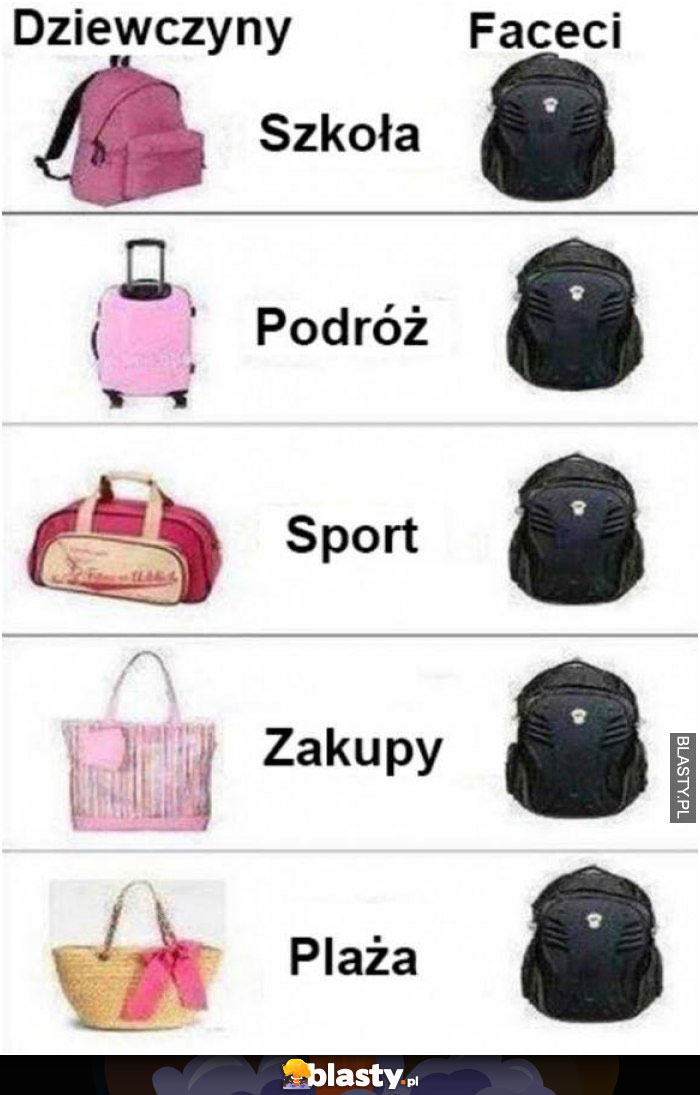The image depicts a Polish meme organized into five rows and two columns, comparing bags for women and men in various categories. Each row showcases different types of bags for women on the left and the same black backpack for men on the right. The bags for women include a pink backpack in the first row, a pink suitcase in the second, a pink duffel bag in the third, a pink tote bag in the fourth, and a tan bag with a pink ribbon in the fifth. Separating each pair of bags is a Polish word indicative of different scenarios or events, including terms like Zuzeni, Fasi, Cola, Podros, Sport, Tsukupi, and Plaza. An additional text, "blasty.pl," is displayed at the bottom of the image, hinting at a website, which possibly compares bags or conveys a humorous comparison. The image's clean, well-centered layout with high contrast colors like black, pink, white, and tan further emphasizes its meme structure.